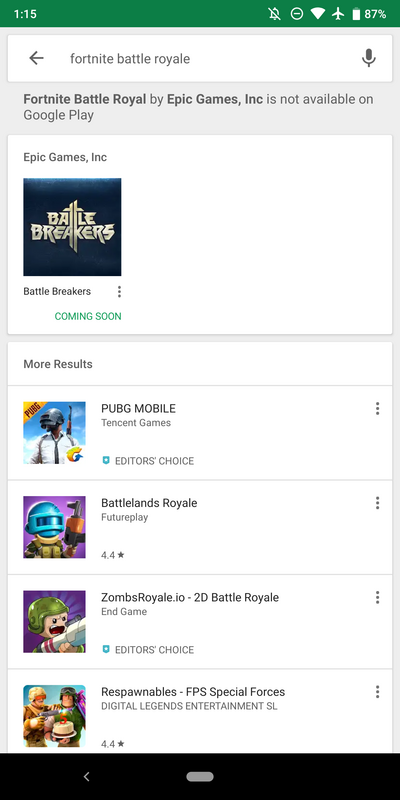The image depicts a search results page that highlights various battle royale games. At the top of the page, the search bar does not specify if the search engine is Google, but "Fortnite Battle Royale" is clearly visible. Below, it indicates that Fortnite Battle Royale by Epic Games Inc is unavailable on Google Play. Below this message is a notification that Epic Games Inc's Battle Breakers is coming soon. The search results feature numerous animated and vividly colored labels for different games. Among these, notable entries include PUBG Mobile, which is marked as an Editor's Choice, Battlelands Royale, Zombie Royale, 2D Battle Royale, and Endgame. Another highlighted game is Respawnables: FPS Special Forces by Digital Legends Entertainment. The page is a vibrant collection of game listings, emphasizing popular and upcoming battle royale titles.